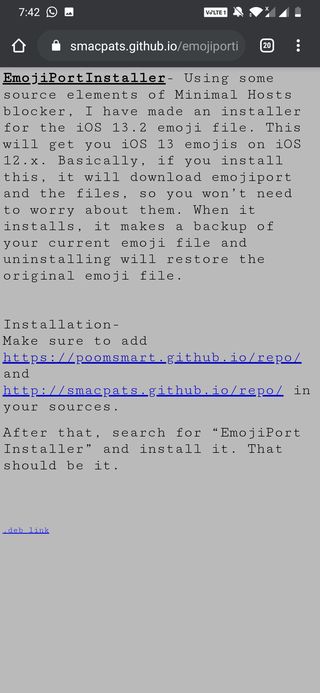The image is a screenshot from a mobile device, as evidenced by the black status bar at the top, which displays the time (7:42), battery level, Wi-Fi signal, and connection icons. The URL bar contains the address "smackpats.github.io/emoji-port" next to a home icon, with a tab indicator showing 20 open tabs, and an options menu represented by three vertical dots.

The main content of the page is a detailed guide titled "Emoji Port Installer" which explains the process to install iOS 13 emojis on devices running iOS 12.x, using source elements from "Minimal Host Blocker." The guide assures users that the installer creates a backup of the current emoji file and automatically restores it upon uninstallation. The installation instructions provided include adding two specified URLs to the device's sources via HTTPS, then searching for and installing the "Emoji Port Installer." The page provides step-by-step details to ensure a smooth and worry-free installation process.